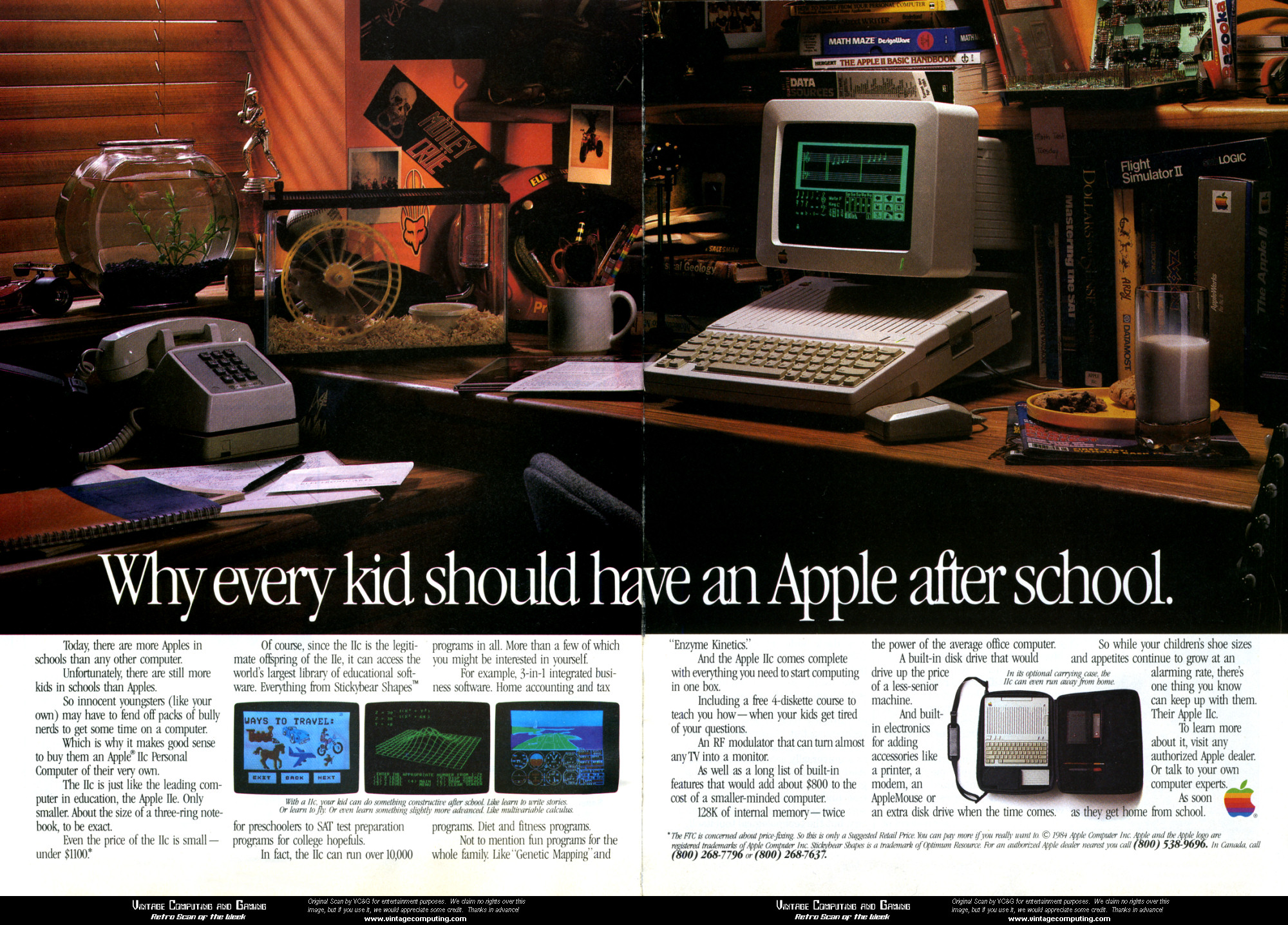The advertisement is a vintage, print spread promoting Apple computers, titled "Why Every Kid Should Have an Apple After School." The scene is set on a rectangular, wooden desk, likely in a child's room or home office. At the centerpiece of the image is a classic Apple computer from the 1980s, featuring an ivory plastic monitor, keyboard, and a triangular mouse. Surrounding the computer are various nostalgic items, including a glass vessel with a hamster wheel, a traditional gray, push-button telephone, and a rounded fishbowl.

Above the computer, on a cluttered bookshelf, are multiple textbooks and games, notably "Math Maze" and "The Apple Basic Handbook." Additional items like a stack of magazines, a yellow plate, and a glass of milk add to the lived-in feel. A white mug filled with pencils, a glass fishbowl, and the rodent aquarium with wood shavings complete the eclectic desktop arrangement.

The advertisement's visual elements are in muted browns, oranges, and rusts, creating a darkened room atmosphere with a spotlight on the silver Apple computer. Beneath the bold, white headline “Why Every Kid Should Have an Apple After School,” there are several paragraphs detailing the benefits and features of Apple products, along with images of monitor screens. The overall composition evokes a sense of nostalgia and the timeless value of Apple technology in education.